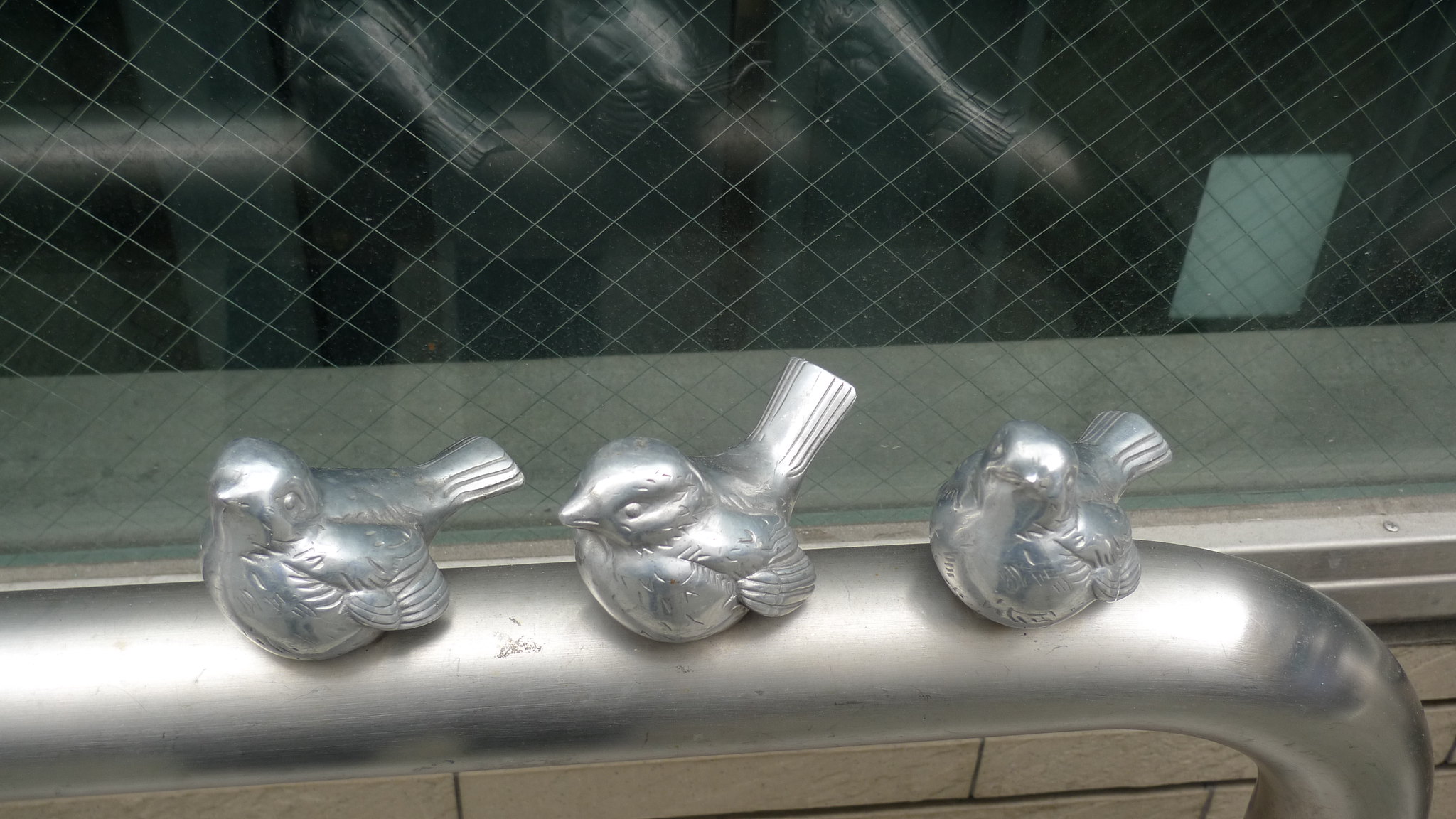This photograph captures a serene and detailed scene featuring three small, silver-colored bird sculptures, each mounted on a sleek, chrome-like metal rail. The birds are aligned in a row, all facing to the left, with the one in the middle looking straight ahead and the outer two tilting their heads upwards. Their design includes intricate feather textures, long tails, tiny beaks, and small, round eyes. The reflective quality of the sculptures matches the shiny rail, suggesting they are fixed to it. 

In the background, there's a window with a distinctive crisscrossing thin white grid pattern embedded in the glass, providing a textured backdrop. The window, likely made to be secure, creates an optical illusion of reflection, giving depth to the scene. The setting includes elements of a brick-built structure, aligning well with the metallic and glass components. This harmonious juxtaposition of materials — metal, glass, and brick — adds a textured and layered complexity to the visual narrative of the image.